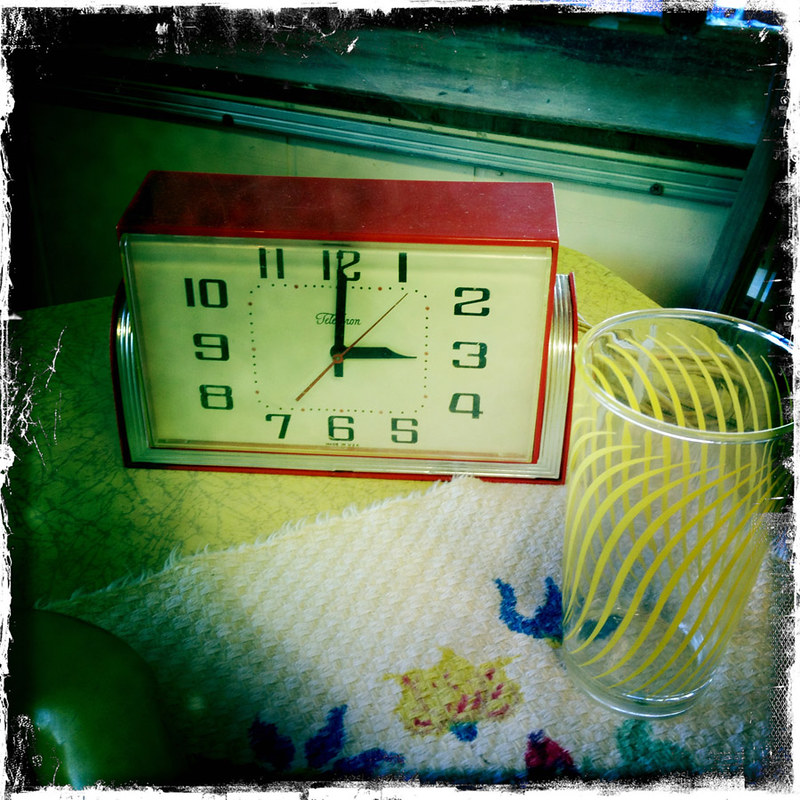In the image, we're presented with a top-down view of a square clock resting on a table. The clock is predominantly red, with red edges and a red top. The numbers on the clock face are arranged as follows: 12 at the top, then 1 through 3 on the right, 4 through 6 at the bottom, 7 through 9 on the left, and 10 and 11 leading back up to 12. The short hand points to 3, the long hand points straight up at 12, and the seconds hand points to 1.

Beneath the clock is a white cloth, casting a shadow on its left side that gives it a greenish hue under the shadow. The cloth features a design incorporating blue, yellow, and red elements. To the right of the clock, there is a glass decorated with a pattern of long, curved yellow lines running from its top to bottom.

In the background, a partial view of a wall and the black frame of a window can be seen, providing context to the placement of the items within a room.